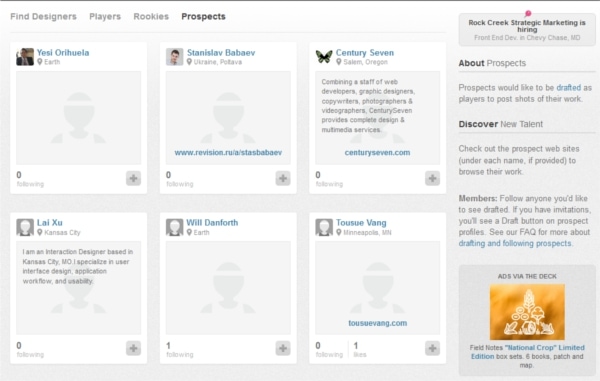The image features a sophisticated layout with a black horizontal line across the top, set against a light gray background. The header text reads, “Find Designers, Players, Rookies,” with the word “Prospects” emphasized in bold black font.

Below the header, the central section of the image is divided into two rows, each containing three vertical segments. These segments initially present an image in the upper left corner of each section, accompanied by a name written in turquoise. Presently, most of these images are blocked off, leaving twelve visible segments in total.

On the right side of the layout, there's a small push pin icon attached to a notification that reads: "Rock Creek Strategic Marketing is hiring." Below this, in light gray font, it specifies the position "Front End Developer," including the location "Chevy Chase, Maryland."

The description area begins with "About Prospects," where "About" is in bold black font and "Prospects" in light gray. This section explains that prospects aspire "to be drafted," with "drafted" highlighted in turquoise. Prospects can post shots of their work, and viewers are encouraged to "Discover New Talent," with "Discover" in bold black font and "new talent" in light gray. It advises viewers to check out prospect websites under each name, if provided, to browse their work.

Additionally, there’s guidance for members: they can follow any prospect they'd like to see drafted. If they have invitations, a draft button will appear on prospect profiles. A final note directs users to the FAQ section, written as “F A Q,” for more details about "drafting and following prospects," with "drafting and following prospects" highlighted in turquoise.

Near the bottom, a light gray box contains a prominent gold rectangle with white text. This section highlights “Fields” in gold font, followed by “Actual Field Notes” in turquoise, and concludes with details about a "National Crop Limited Edition Box Set" in black font, noting it includes six books, a patch, and a map.